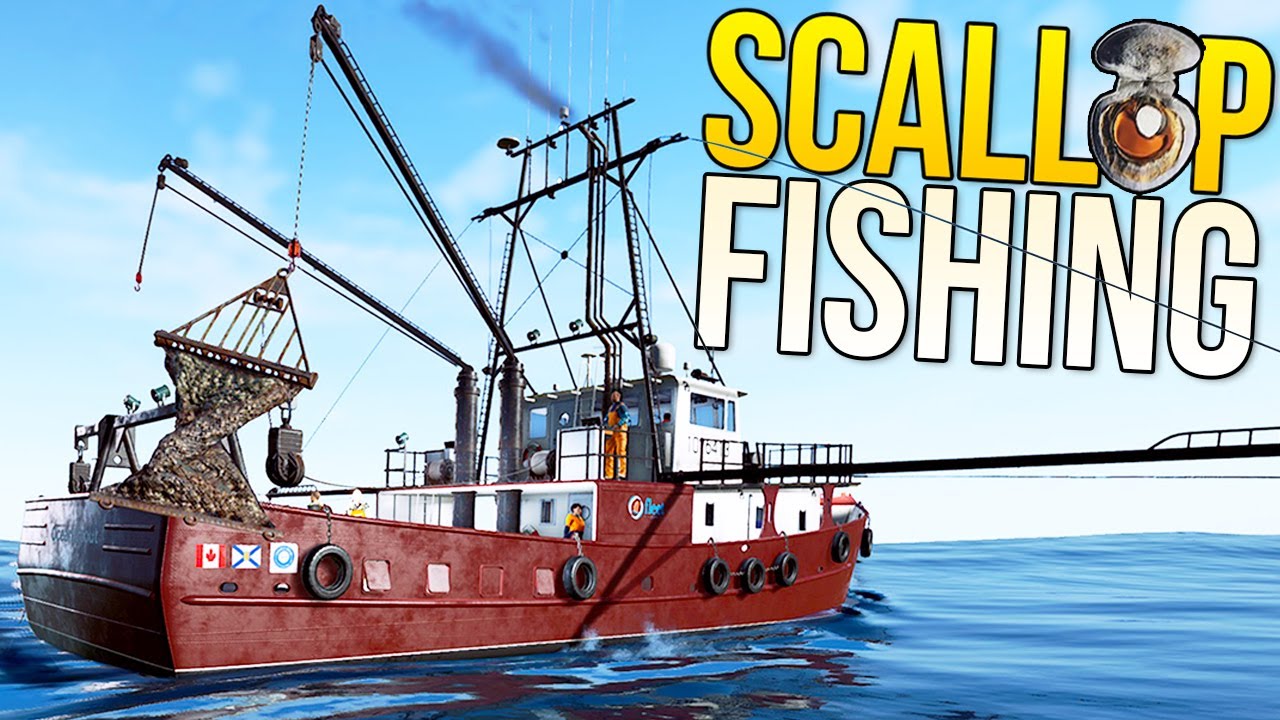The image features a modern red fishing boat engaged in scallop fishing on a clear, expansive blue ocean with no other visible landmarks, clouds, or boats. The boat’s upper deck is predominantly white, contrasting with its red hull, which is lined with fenders and lifesavers. Three people in yellow coveralls or shirts are visible on the boat, operating multiple cranes and pulleys that are lifting a large net full of scallops from the water at the back left side. Prominent in the upper right-hand corner of the image is the text "Scallop Fishing" where "Scallop" is rendered in large yellow letters with an O replaced by an open scallop shell graphic, while "Fishing" is in white letters. Additionally, a small Canadian flag is noticeable at the rear of the boat. The overall composition suggests it could be used as a postcard or a YouTube interstitial graphic.